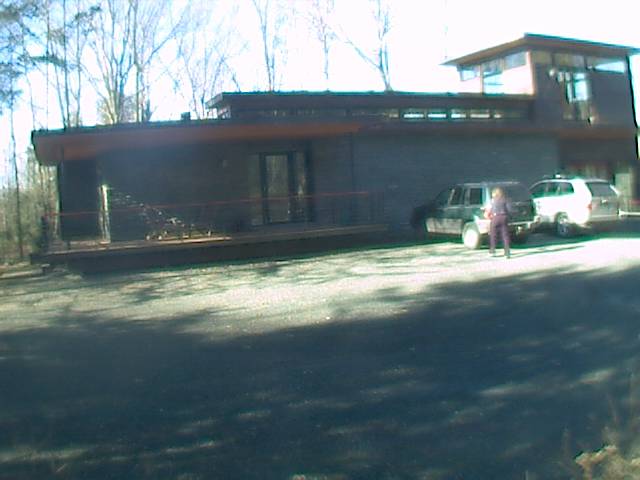A detailed image description:

The image showcases a rectangular, dark brown building with a front porch. The structure features a unique three-tiered roof design and windows that are situated high, near the ceiling, around the building. The scene is set on a blacktop parking lot, with two station wagons parked in front of the building. It is daytime, as evidenced by the sunlight reflecting and casting shadows on the ground. In the background, a tree-laden area is visible, with trees that have some leaves remaining, suggesting the photo was taken in late fall, early winter, or early spring.